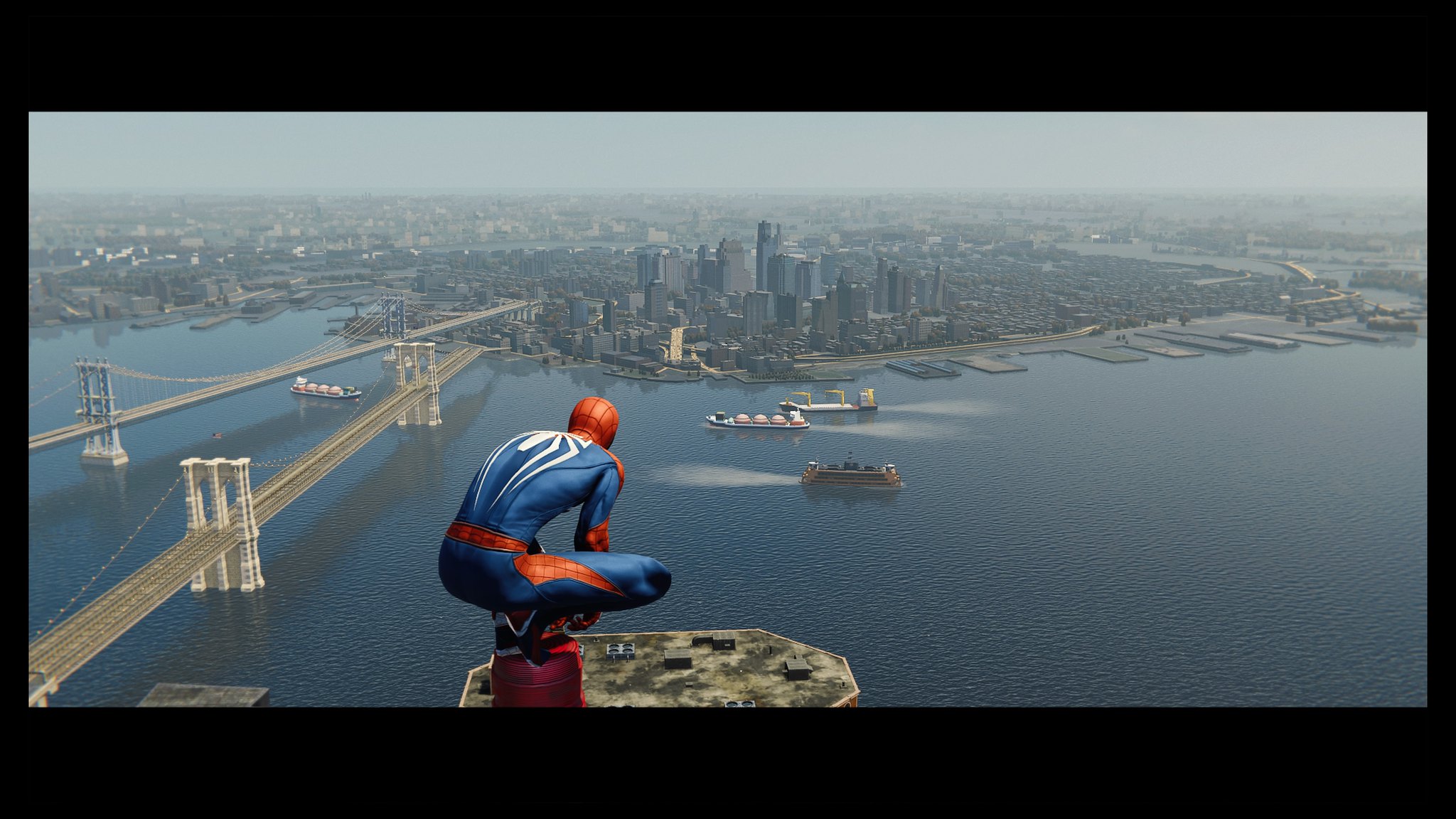The image depicts Spider-Man crouched on top of a red cylinder situated on a flat, dirty white platform, high above a sprawling, slightly foggy city that could be either New York City or Gotham City. Spider-Man's costume features a hood or mask that is red with webbing details, along with a navy blue bodysuit adorned with a white spider emblem on the back and red streaks on the legs and waist. To the left of Spider-Man, there are two long bridges stretching across a river, likely Hudson Bay, with multiple boats, including flatboats and a ferry, navigating in both directions. The densely packed skyscrapers fade into the light blue sky at the horizon, creating a misty, atmospheric effect that blends the buildings into the background. The image is bordered by a thick black matte, suggesting it might be a widescreen movie screenshot.